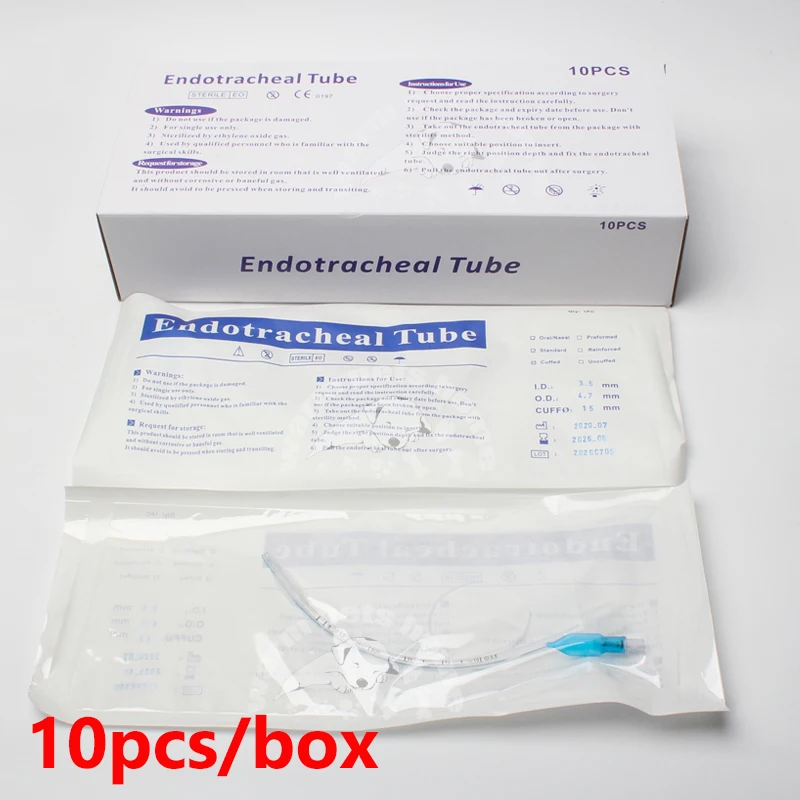The image displays a detailed presentation of an endotracheal tube product package. Set against a grayish-white background, the picture is organized into three stages. At the top, there is a simple white box with purple writing indicating it contains "Endotracheal Tube" and specifies "10 pieces" in the top right corner. The middle section shows an individual tube that has been removed from the box, laying flat with blue writing identifying it as an endotracheal tube. The final stage at the bottom illustrates the back side of an individual tube package, which is clear plastic, allowing a view of the transparent tube inside with a hint of light blue at its tip. In bold red text at the bottom right corner, it again notes "10 pieces/box." Overall, the image provides a comprehensive view of the product box, an individual packaged tube, and the clear packaging revealing the tube inside.